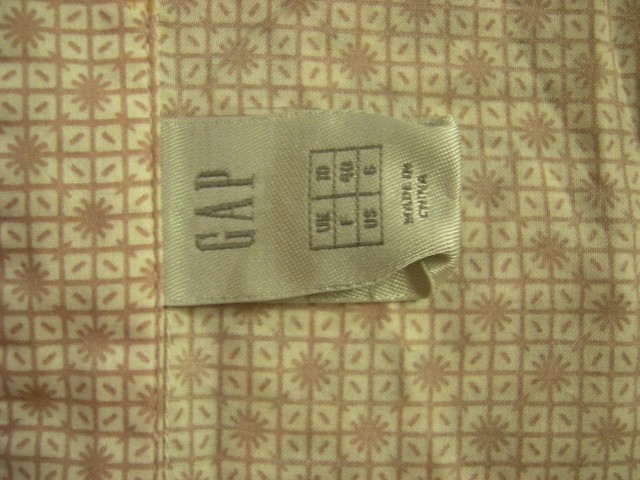This is a color photograph showcasing an up-close view of a tan fabric with a detailed checkerboard pattern composed of horizontal and vertical brown lines. Within some squares of the pattern, delicate designs such as stars, tiny flowers, and crisscrossing lines enhance the visual texture. The fabric stretches across the entire frame, from left to right and top to bottom. At the very center of the image is a vertically oriented, bronzed tag affixed to the garment. The dimly lit photograph captures the tag's capitalized, vertical letters "GAP," followed by a grid detailing sizing information, with the US size 6 being legible. Below the size information, in vertical lettering, it states "Made in China." The image is slightly out of focus, adding a subtle blur to the intricate details.